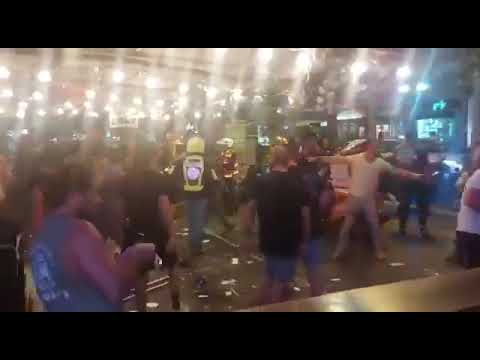The image depicts an indoor scene, possibly of a party or emergency event, but is notably blurry and obscured by bright lighting. In the foreground, a man with dark, pulled-back hair and wearing a sleeveless shirt is visible. Central to the image are individuals who may be wearing neon yellow and black jackets, suggestive of firefighters, implying a possible emergency situation. Bright, elongated lights from the ceiling cast a dazzling glare that further washes out details. Amidst the crowd, a man in a white shirt with outstretched arms appears to be directing or guiding people, while others in black shirts and blue shorts mill about in what seems to be a large, columned room. The overall effect is one of confusion and urgency, amplified by the overwhelming bright lights and the multitude of indistinct figures.